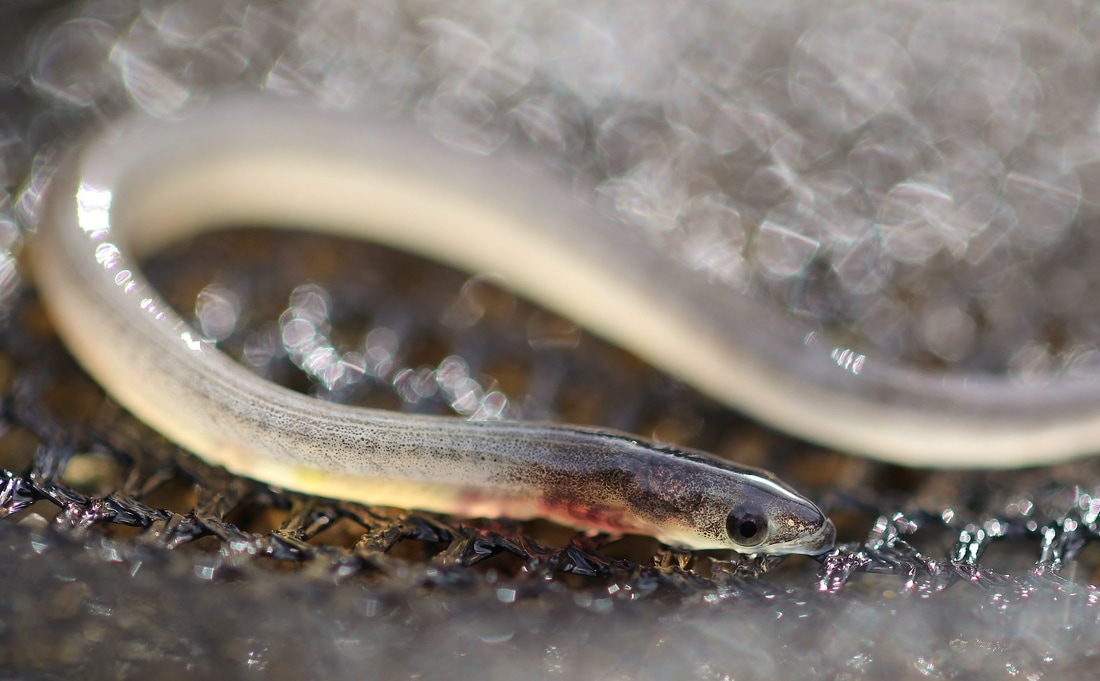This is a detailed close-up photograph of a small, possibly juvenile, snake with an elongated, thin body. The snake appears translucent, with a combination of white and clear skin that allows a faint view of its internal structures, including some reddish and black coloring. Its head, adorned with black and gray dots, is prominently visible. The snake's right eye is clearly seen, round and black, giving the creature a somewhat beady appearance. The mouth is closed, and the head, along with most of its neck and body, is in focus. However, the middle of the body appears more blurred, probably due to depth of field in the photograph. The snake is laying on a surface that is shiny and shimmery, resembling ice or crystal-like material, adding to the ethereal quality of the image.